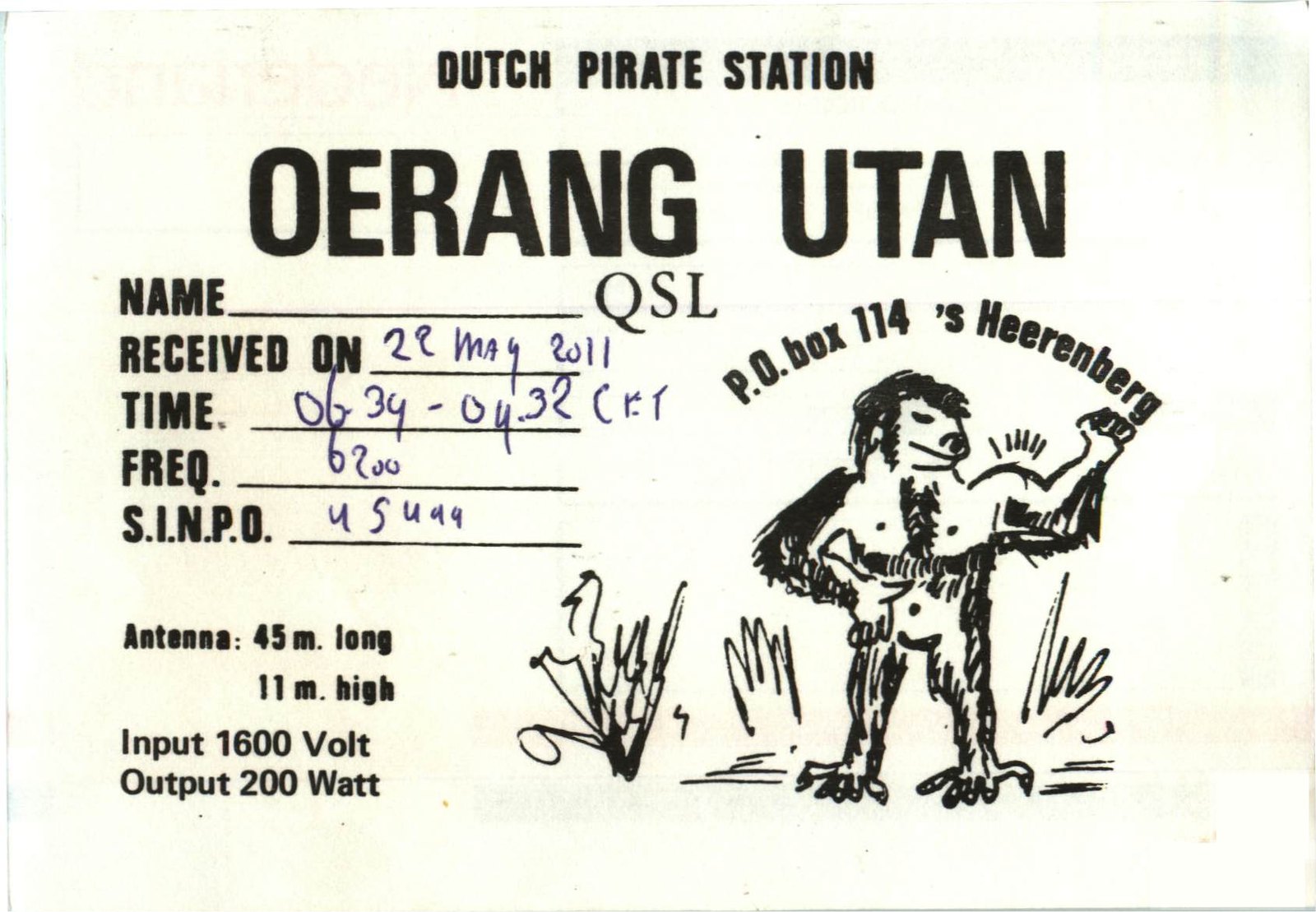The image is a hand-drawn poster or card with a white background and black lettering. At the top in bold, capitalized print, it reads "DUTCH PIRATE STATION." Below that, in large, capitalized letters, "O-E-R-A-N-G-U-T-A-N" is inscribed, with "P.O. Box 114, S-H-I-R-E-N-BurG" written above the drawing. On the bottom right, there is a sketch of a very hairy, muscular figure, likely an orangutan, standing in grass and making a muscle with lines above his bicep. The figure, possibly depicted with exaggerated features resembling bird-like feet, adds to the whimsical quality of the artwork.

Underneath the orangutan's name, several lines of text provide technical reception details:
- "Name: __________"
- "QSL"
- "Received On: 22 May 2011" (handwritten in pen)
- "Time period: 0634-0932 CET"
- "Frequency: 6200"
- "SINPO: 45444" (or potentially "4544UAA")
- "Antenna: 45-M long, 11-M high"
- "Input: 1600 volts, Output: 200 watts"

The piece serves as an intricate combination of whimsical art and detailed technical information, representing a broadcast from a Dutch pirate radio station.